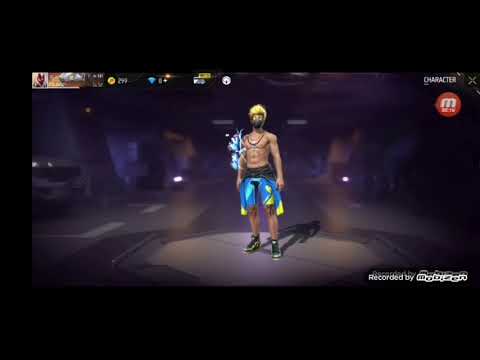This screenshot of a video game captures a central shirtless male avatar with a tan complexion. The avatar sports a black beard and short, blonde hair or possibly a yellow helmet. He dons a distinctive necklace and black high-top sneakers. The blue, black, and yellow shorts he wears are complemented by additional garments that suggest either a wetsuit with the top portion hanging down or decorative feathering on his right arm. The scene hints at a dark setting illuminated by a spotlight, with indistinct lights in the background. Notable on the screen, the lower right corner contains the white text "recorded by M-O-B-I-Z-E-N." Meanwhile, the upper right corner features the word "CHARACTER" in all capital letters with an 'X' beside it, and just below it, a red circle with an 'M' inside.